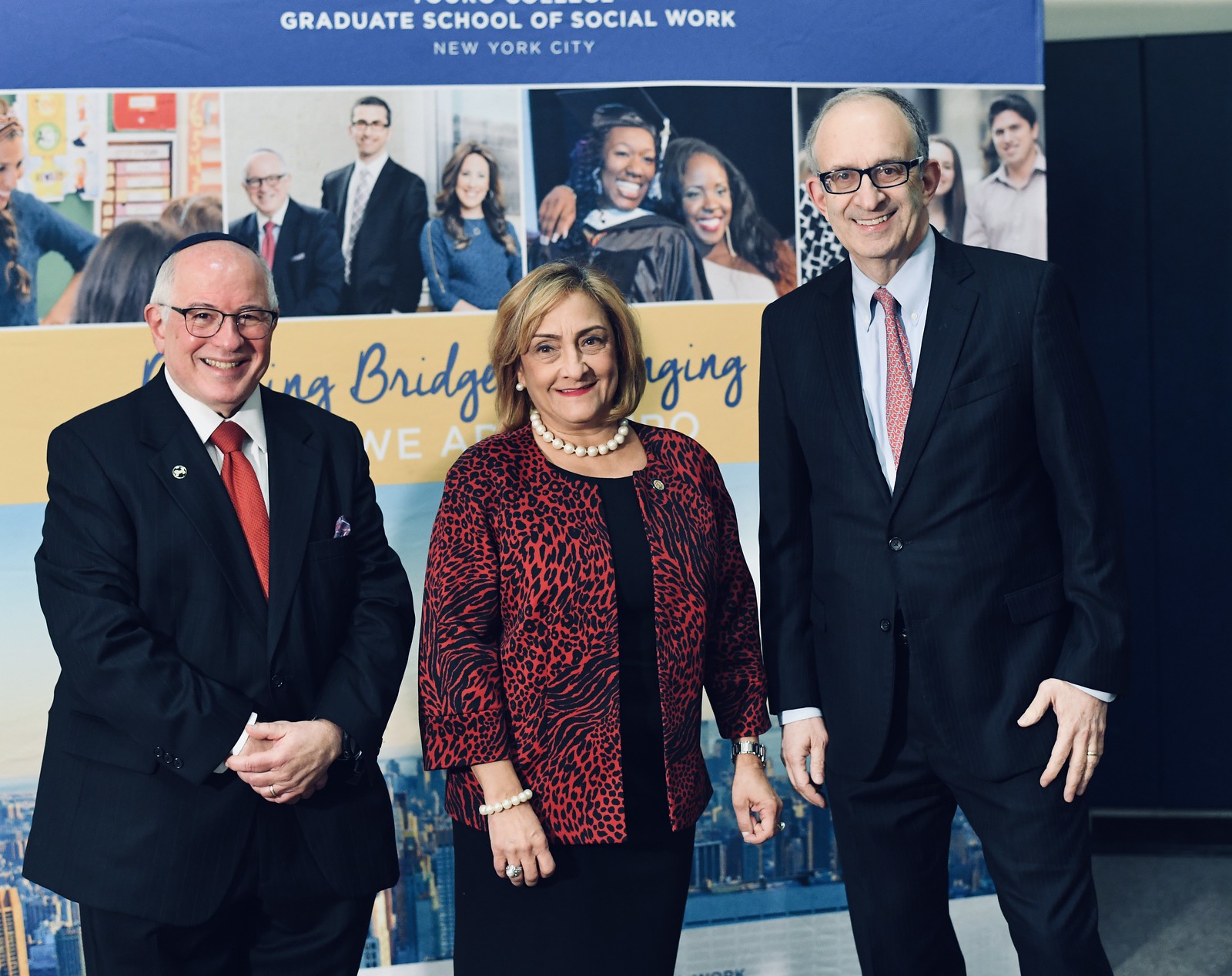The image showcases three older individuals standing in front of a large banner for the Graduate School of Social Work in New York City. The banner, with a blue background and images depicting various people in educational and graduation scenarios, features the New York City skyline at the bottom. 

On the left is an older Jewish man, identifiable by his yarmulke and bald head. He is smiling and wears glasses along with a traditional black pinstripe suit, a white dress shirt, a red tie, and a blue or purple handkerchief peeking from his pocket. His hands are clasped in front of him, and he has a round lapel pin and a wedding ring.

In the center stands an older woman with shoulder-length auburn hair, adorned with pearls—pearl earrings, a pearl necklace, a pearl bracelet on her right wrist, and a ring with a pearl. She is dressed in a black dress topped with a red and black leopard print jacket. Her left wrist sports a watch and another ring.

To the right is the tallest individual of the trio, another older man. He is wearing black thick-rimmed glasses and smiles warmly. His attire includes a dark pinstripe suit, a light blue dress shirt, a red and white speckled tie, and a wedding ring. All three exude a sense of ceremony and formality, consistent with the academic event they are attending.